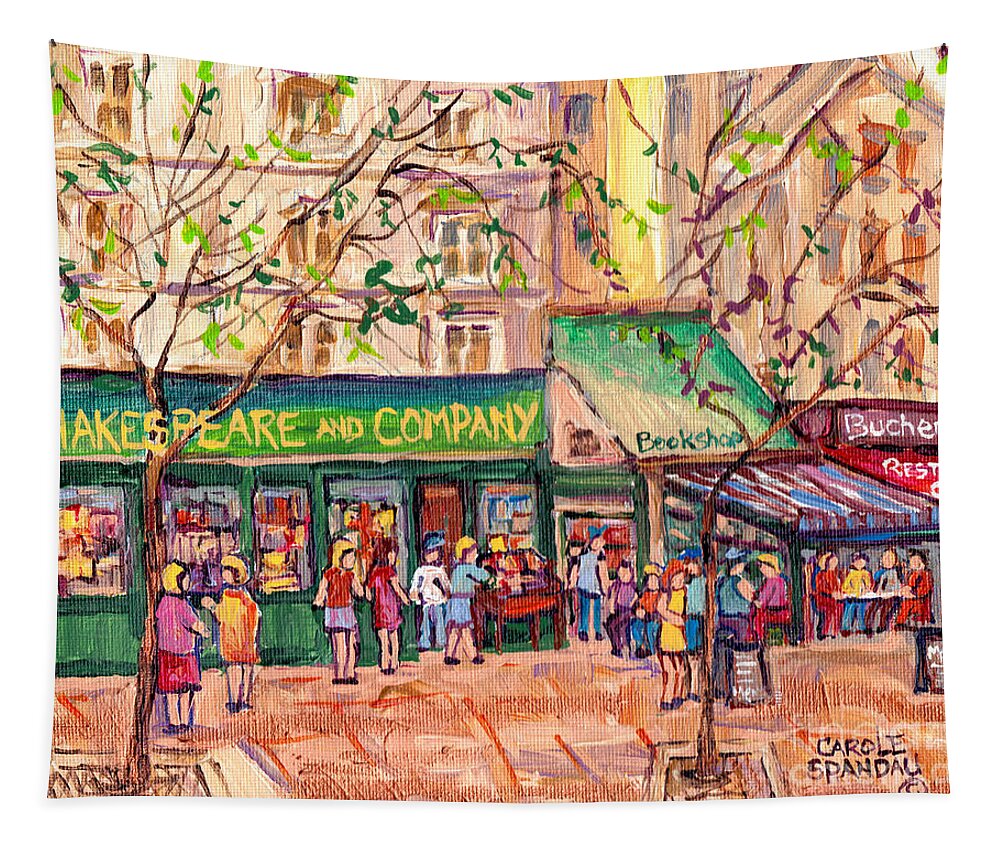This detailed painting by Carol Spandau depicts the bustling scene in front of the famous Shakespeare and Company bookstore in London. Painted with thick brush strokes on canvas, giving a rich texture, the artwork captures a crowded street with numerous people whose faces are indistinct. The bookstore, situated in a green three-story building with "Shakespeare and Company" prominently displayed, anchors the left side of the painting. Adjacent to it is another bookshop with a green awning labeled "Bookshop." 

A vibrant café with a blue and red awning sits to the right, its diners enjoying meals at tables close to the sidewalk. Both the bookshop and the café feature sandwich boards in front, advertising their offerings. In front of these buildings, two sparse trees with green leaves are rooted in the sidewalk. Above and behind the street scene, additional buildings with numerous windows fade into the background, contributing to the depth and urban feel of this colorful oil painting. The street beneath is painted in shades of brown, enhancing the earthiness and bustle of this iconic location.